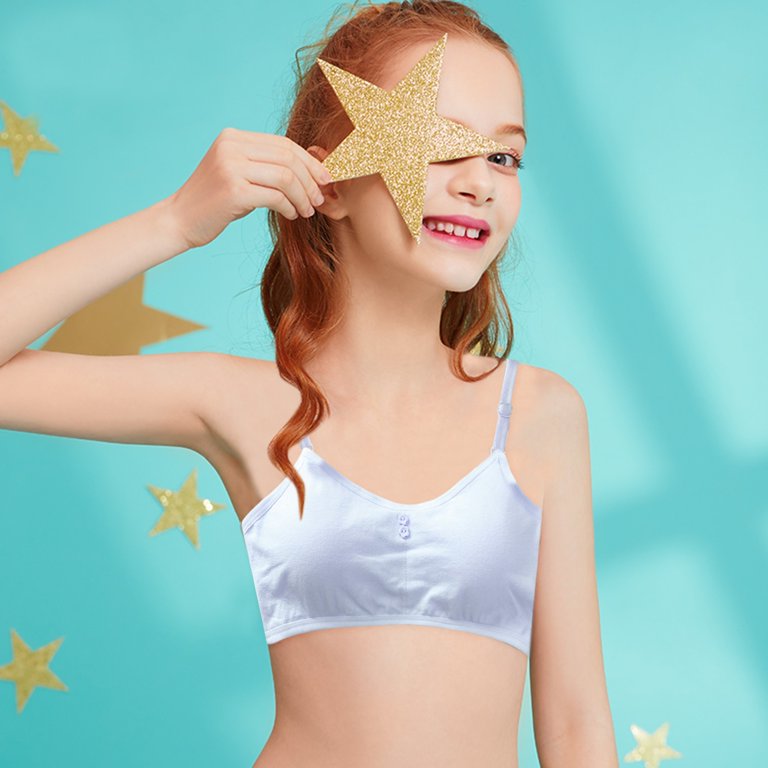This photograph captures a young girl, approximately 6 to 8 years old, with vibrant red hair cascading below her shoulders. She stands against a light blue background adorned with both gold and silver stars, some glittery and some flat. She holds a large gold glittery star over her left eye, playfully peeking out with a bright smile that reveals a charming gap between her teeth. The girl's complexion is very pale, complementing her strawberry blonde hair, red eyebrows, and strikingly fair blue eyes. She is dressed in a light blue, possibly satin, garment that looks like a cropped top or a training bra, adorned with two star or flower-shaped buttons. The photograph is taken from waist up, creating an endearing and whimsical scene that appears either styled for a playful photo shoot or part of a modeling set.